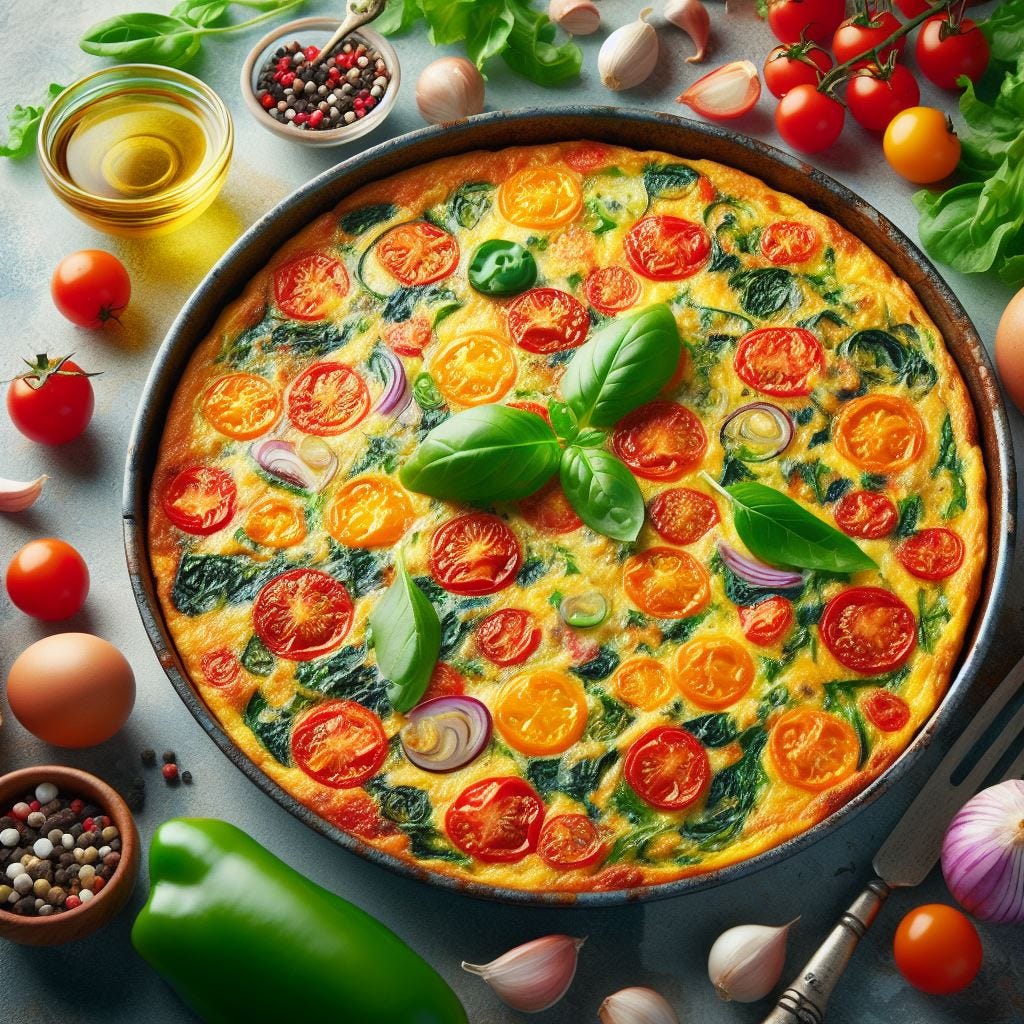This close-up photograph presents a beautifully arranged brunch scene centered around a savory, golden-baked quiche housed in a round metal baking pan. The quiche is adorned with vibrant, sliced cherry tomatoes, chopped red onions, and ample spinach, all set within a rich, egg-based filling speckled with melted yellow cheese. In the center and sporadically across the quiche, fresh basil leaves add a touch of green flair. Surrounding the pan, an appetizing array of ingredients contributes to the rustic aesthetic: scattered cherry tomatoes, garlic cloves, a large green pepper, whole eggs, reddish-purple onions, and a jalapeño pepper. Complementing these are small bowls containing olive oil and a variety of colorful peppercorns. A silver fork adds practicality and finish to the scene, placed just outside the lower right edge of the pan.